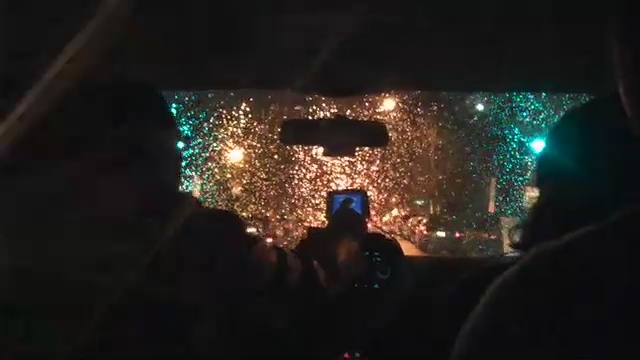A photograph taken from the backseat of a car offers a view looking forward through a rain-streaked windshield at nighttime. Raindrops scatter and cling to the glass, illuminated in a kaleidoscope of colors from various light sources. Some raindrops glimmer in a soft green hue, reflecting the glow of a traffic signal, while others shimmer in golden tones, cast by nearby streetlights. The ambient light creates an atmospheric mood, emphasizing the contours of both the driver and the passenger, whose outlines and headrests are discernible against the dimly lit interior of the vehicle. The driver’s hand is mid-motion, tapping on the car's navigation screen, hinting at the journey ahead. The interplay of light and rain creates a mesmerizing and almost cinematic scene, capturing a fleeting, intimate moment within the confines of the car.